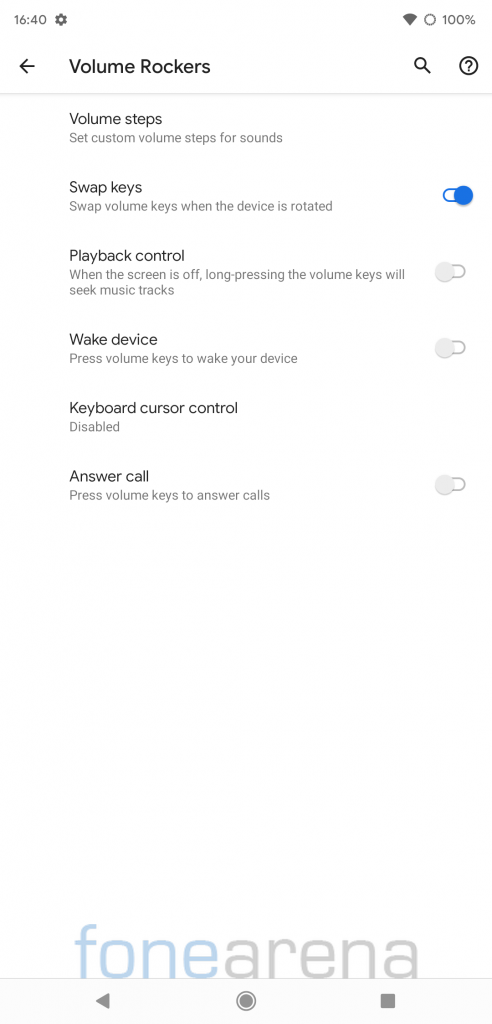A detailed screenshot description of a smartphone settings screen:

The screenshot shows a smartphone screen with a white background. On the top-left corner, the time reads "16:40" in black text. Next to the time, there's a gear icon, indicating settings. On the top-right, there are three icons: a Wi-Fi signal icon, a circle, and a "100%" battery life indicator, all in black.

Beneath this header, the screen is divided by a horizontal gray line. Below this line, the top of the settings section starts with bold, black text stating "Volume Rockers." To the left of this label is a left-pointing arrow, and to its right, there are a magnifying glass icon and a circular icon with a question mark inside.

Following this, there are six settings options listed in bolded black font:
1. **Volume steps** 
2. **Swap keys** 
3. **Playback control**
4. **Wake device** 
5. **Keyboard cursor control**
6. **Answer call**

Underneath each setting name, there is a short description in smaller, gray font. To the right of the "Swap keys," "Playback control," "Wake device," and "Answer call" settings are slider switches. The "Swap keys" slider is lit in royal blue, indicating that it is turned on. The remaining sliders are grayed out, showing that they are turned off.

The bottom portion of the screen displays additional gray space below the "Answer call" setting. At the very bottom of the screen, there is the text "Tepsys's phone arena," with "Tepsys's phone" in a light blue color and "arena" in gray.

Finally, at the bottom edge of the screen, there are three navigational icons: a left-pointing triangle on the left, a circle in the center, and a square on the right.

This detailed description provides a clear and comprehensive understanding of the smartphone settings screen layout.